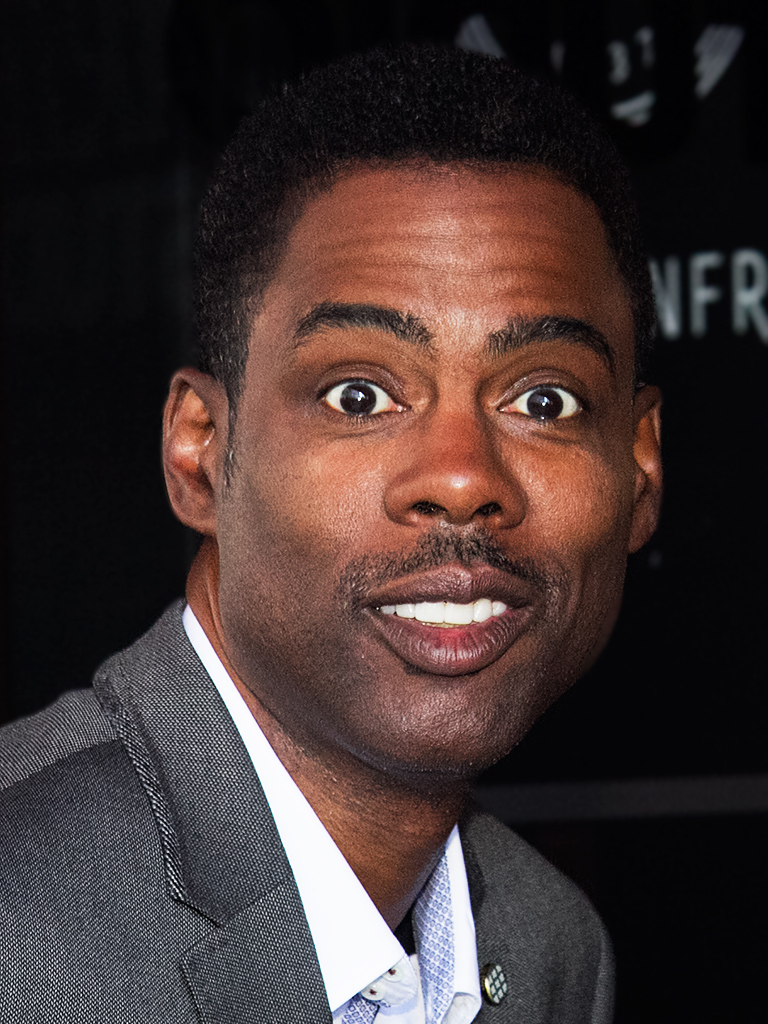This image is a close-up photograph of an African-American male comedian with dark brown skin and a one-inch curly afro. He has thick, curvy eyebrows and dark brown eyes. His expression is one of surprise, with wide-open eyes, and he is smiling slightly with his mouth open but his teeth closed. He features a tiny mustache with clean-shaven sideburns and a little bit of stubble.

He is dressed in a light gray tuxedo paired with a light bluish dress shirt and what appears to be a white tie, though the tie is partially obscured at the bottom of the image. On the right side of his suit jacket, near the top, there is a circular pin or badge made of metal or plastic.

The background is entirely black and features incomplete white text, where the letters "NFR" are partially visible. The man’s body is angled to the right, but his head is turned to look directly at the camera, suggesting this photo was taken at an event, though the specific details of the setting are unclear.